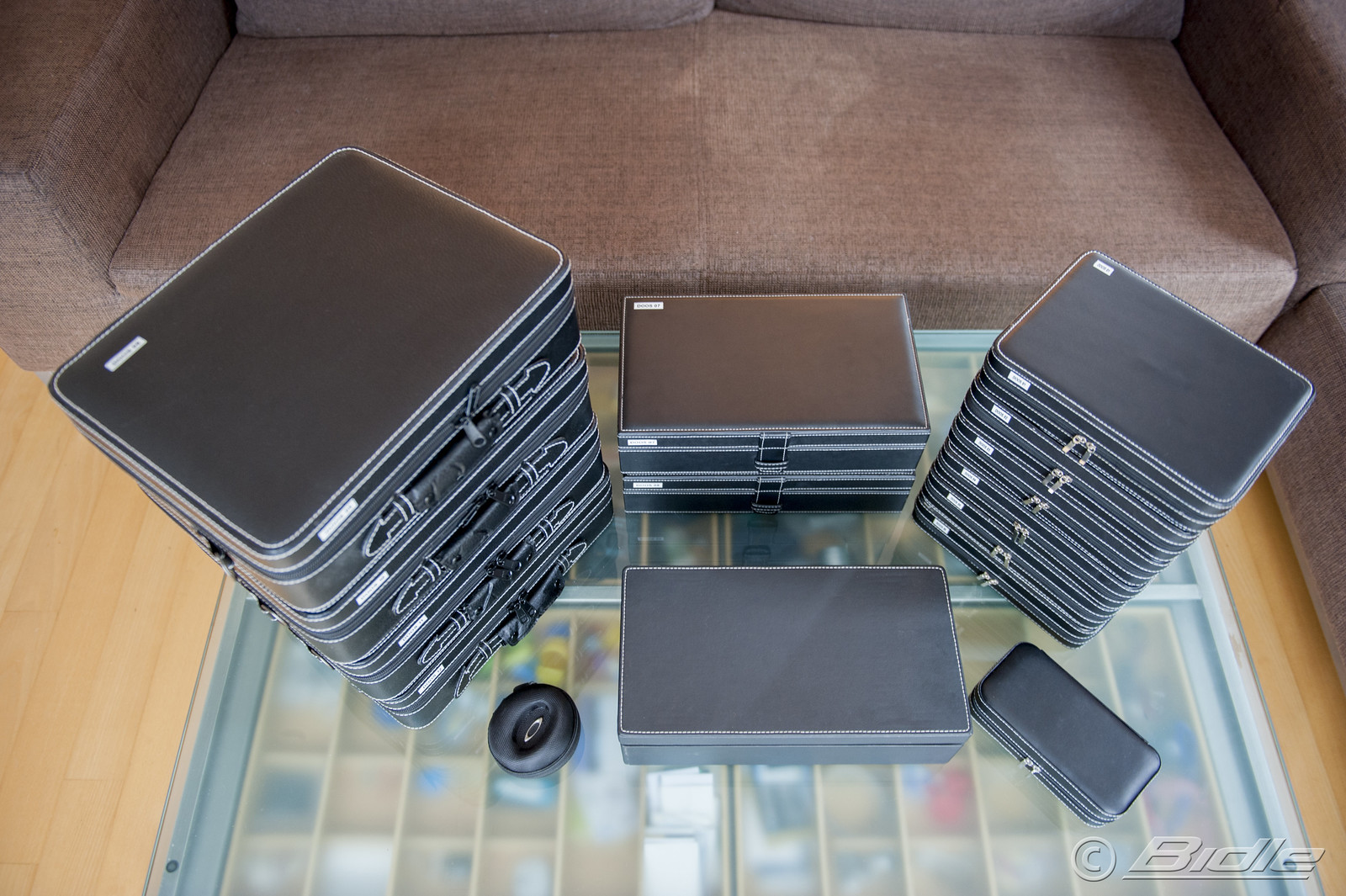This detailed image showcases an assortment of small black leather cases meticulously arranged on a glass table with a clear surface and square patterns. The table stands on a light wooden floor, framed by a gray couch with soft cloth cushions. The black leather cases, which feature white thread borders and black handles, vary in size and shape. On the right side of the table sits a small black leather case, resembling an eyeglass case, next to a larger rectangular black leather case. Further left, there is a small round headphone earpiece. In front of the earpiece, approximately four or five similar rectangular black leather cases are stacked on top of each other. The middle of the table has two similar black leather cases standing on one another, while to the right of these sits a tall line of six smaller rectangular black leather cases. Below this tall stack, a small black rectangular purse or satchel is visible. There is also mention of a big plastic-covered box with various compartments, but it is not clearly depicted in the image.